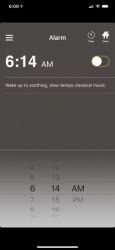The image features a primarily black, blurry background with various elements scattered across it. In the upper left-hand corner and top portion of the image, there are white icons typically associated with a mobile device's status bar. Among them, there is a white bar indicating the battery level, which appears mostly full, a triangle likely representing the Wi-Fi signal, and some other unidentified white elements.

A pop-up overlay dominates the middle of the image, transitioning in color from dark gray at the top to almost white at the bottom. The upper section of this pop-up is blurry but includes three horizontal white lines, possibly representing a menu or settings icon. Below these lines, there appears to be an alarm icon, followed by a white circle and an icon resembling a house.

In the middle of the pop-up, a white timestamp reads "6:14 a.m." in a white font. Adjacent to this timestamp is another white circle, which may be connected to an oval shape, though it's not entirely clear due to the blurriness. Some unidentifiable white elements are present in this section as well.

Toward the lower part of the pop-up, it is evident that the user has selected a specific time setting, as indicated by a black "6," "14," and "a.m." The space between the elements suggests a separation of functions or selections within the pop-up.